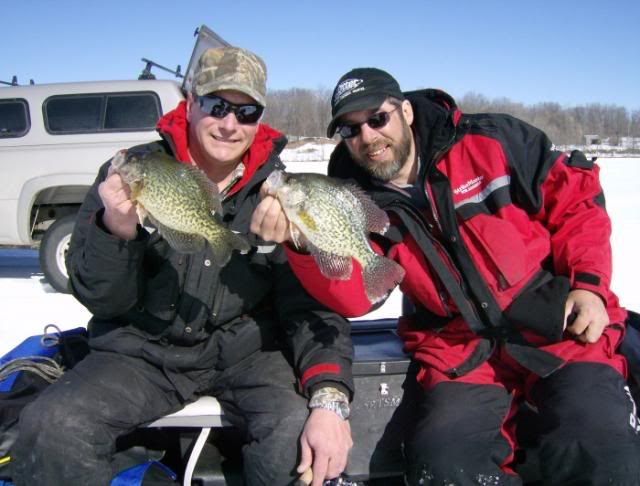In this outdoor scene, two men are proudly displaying their freshly caught fish against a snowy backdrop, suggesting they have been ice fishing. Both are sitting on a bench, dressed in red and black winter jackets with snow-tight black pants, and wearing sunglasses. The man on the left sports a camouflage cap and black sunglasses, while the man on the right, who has a beard and mustache, wears a white and black hat. Surrounding them are trees under a clear, sunny blue sky, and a silver or white truck with a bed cap is visible in the background. The image has text across the middle reading "photo bucket" with the service's logo, and a lower band that states, "protect more of your memories for less."